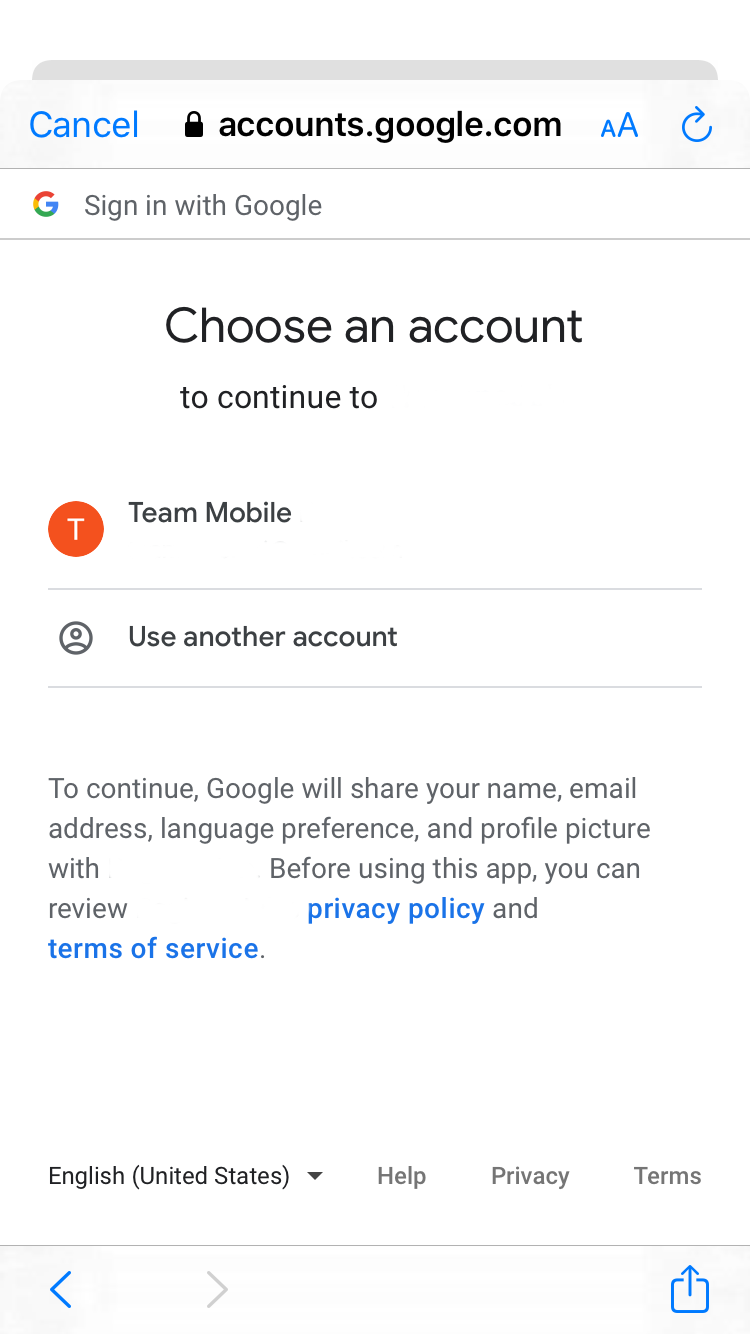The image is a mobile phone screenshot showcasing a Google login page. The web address, "googleaccounts.com," is clearly visible at the top. The page is designed specifically for signing in with a Google account on a mobile device. Below the web address, a header reads "Sign in with Google," followed by a prompt "Choose an account to continue to." The account options displayed include a placeholder labeled "Team Mobile," suggesting it may be a dummy or template account. Below this option, there is a link that says "Use another account" for users who prefer to log in with a different Google account.

Further down, a message informs users that to proceed, Google will share their name, email address, language preference, and profile picture with the service. Certain parts of this message are blanked out, presumably to omit sensitive information. The message also mentions that users can review the privacy policy and terms of service before proceeding.

At the very bottom of the screenshot, the language setting "English (United States)" is displayed, along with links to "Help," "Privacy," and "Terms." Visible as well are the phone's navigation buttons for "Back" and "Forward," indicating the screenshot was taken from an active session.